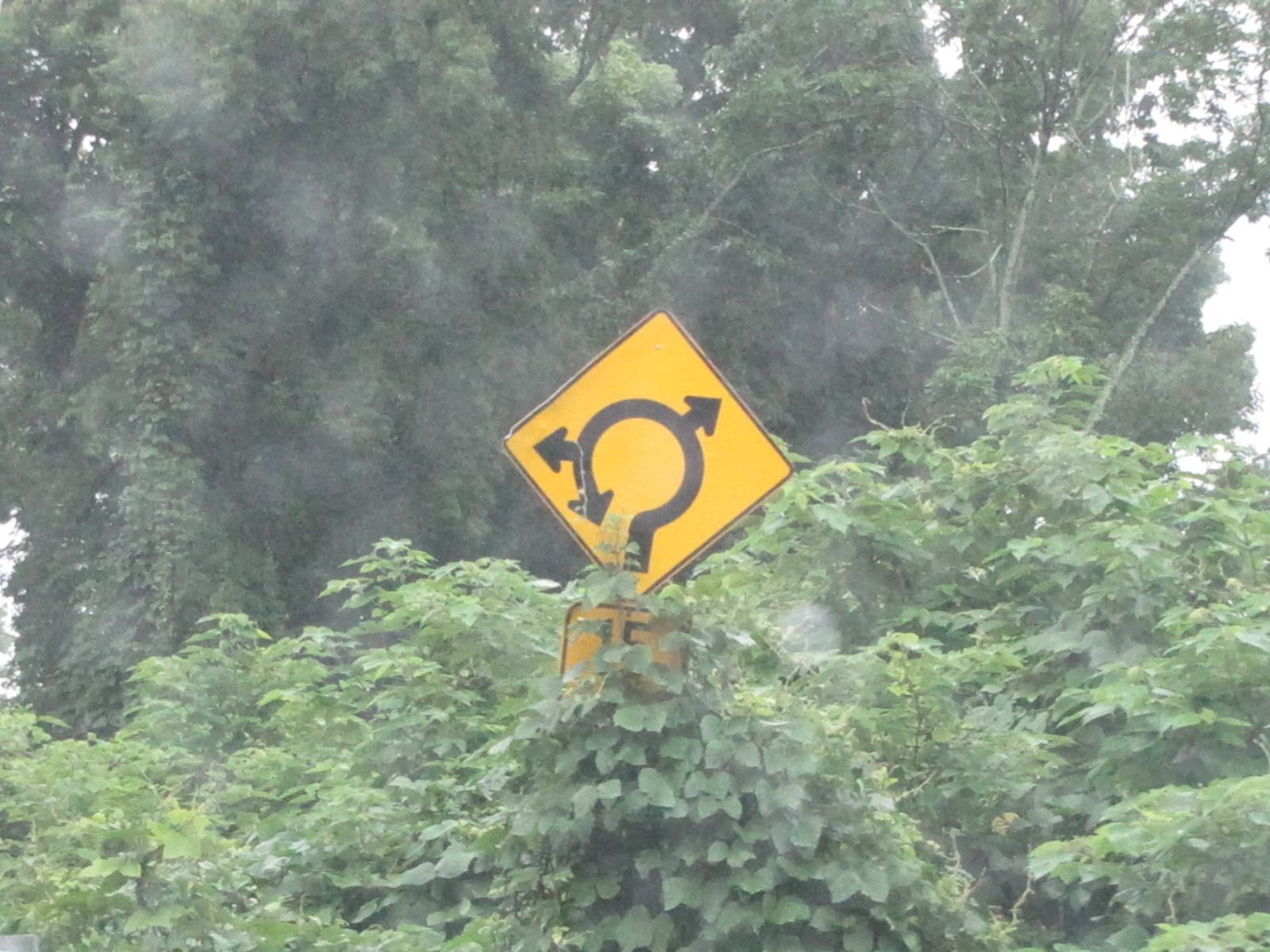The image depicts an outdoor scene dominated by a diamond-shaped, yellow street sign with a roundabout symbol. The primary focus of the sign is a curved, circular line with an arrow at the end, alongside two additional arrows branching off to the left and top right, indicating a roundabout ahead. Dense green bushes and vines have partially overgrown the sign, and another yellow sign below it is mostly obscured, though it hints at a possible numeric designation, like "15." The background features towering, leafy trees and a light gray, hazy sky, giving the photo a somewhat dusty or dirty appearance.